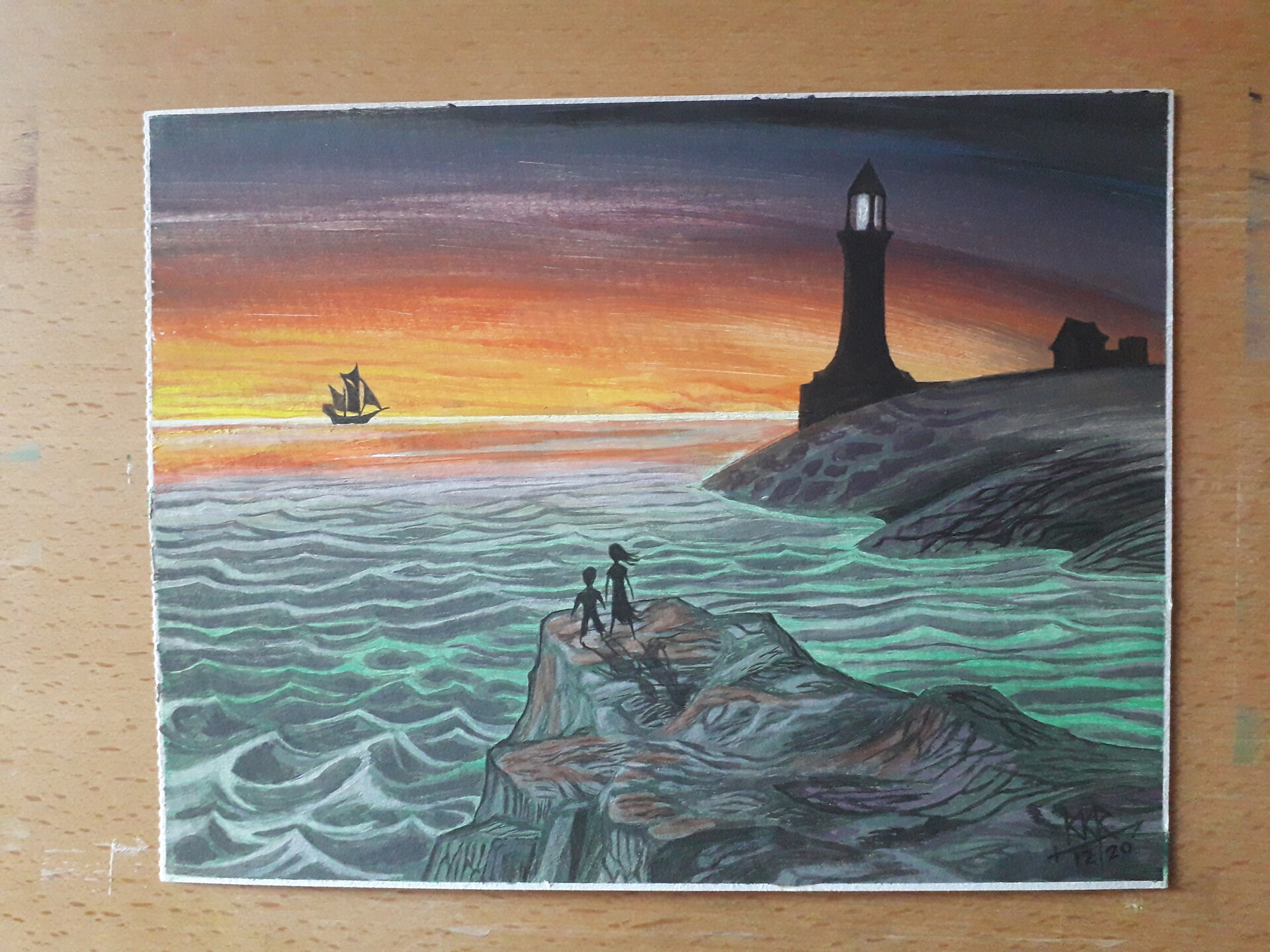This image captures a photograph of detailed artwork, possibly a drawing or a painting, set against a pine wood background, potentially taped down. The vivid scene depicts an ocean view at sunset, with the sky transitioning from yellow and orange hues to dark purples. Central to the artwork are two children, a boy with short hair and a slightly taller girl with long hair, standing on a rock cliff. They appear to be silhouettes, possibly holding hands, evoking a sense of vulnerability as they gaze out over the waves. To the right, a lighthouse stands on a separate cliff island, accompanied by a small house. A sailboat, dark in color, is visible near the horizon where the sun is setting. The tumultuous sea is painted with gray and green waves, adding depth to the scene. The initials "KKR" and the date "12-20" are visible in the bottom right-hand corner of the artwork.